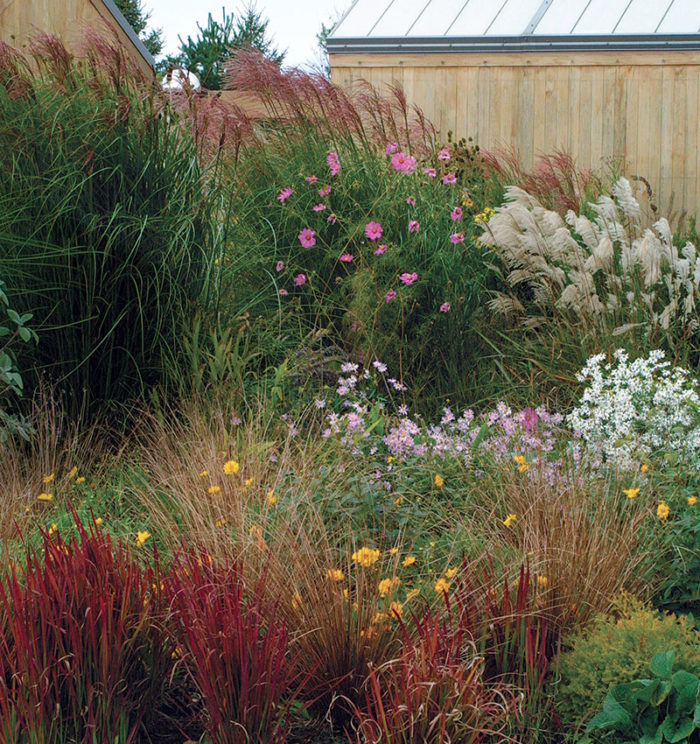This outdoor photograph captures a vibrant, lush garden set against a backdrop of wooden structures with blue slatted and light metal roofs, under a nearly white sky. The expansive garden is predominantly filled with an array of tall, colorful grasses and wildflowers, evoking the feel of a wild desert flower bed. In the forefront, reddish-maroon foliage spikes up from the ground, adding a striking contrast. Tall green grasses with brown tips intermingle with flowers of various hues—light purple ones sparingly appearing amidst the greenery, clusters of bright yellow blooms, and sporadic small white flowers. Among the foliage, some grasses stand out with fluffy white and dark purple tips. Centrally located, two green shrubs enhance the garden's richness, one adorned with hot pink flowers and the other with long, thin leaves. The intricate layers of diverse plant life create a textured, colorful scene, merging seamlessly with the contrasting wooden structures in the background.